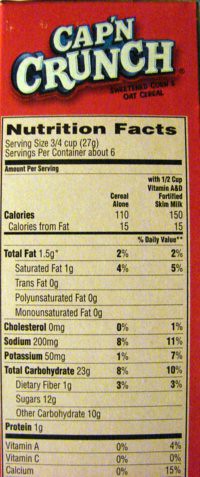This image depicts the side panel of a Cap'n Crunch cereal box. At the very top of the panel, the Cap'n Crunch logo is prominently displayed. Below the logo, there is a section containing nutritional information. This section features a vertically-oriented rectangular box labeled "Nutrition Facts." Key details include a serving size of 3/4 cup and approximately six servings per container. It also lists the caloric content, which is 110 calories per serving or 150 calories when combined with 1/2 cup of milk. Additional nutritional details include 15 calories from fat, a total fat content of 1.5 grams, and 1 gram of saturated fat. The panel provides essential information for consumers seeking to understand the nutritional value of the cereal.